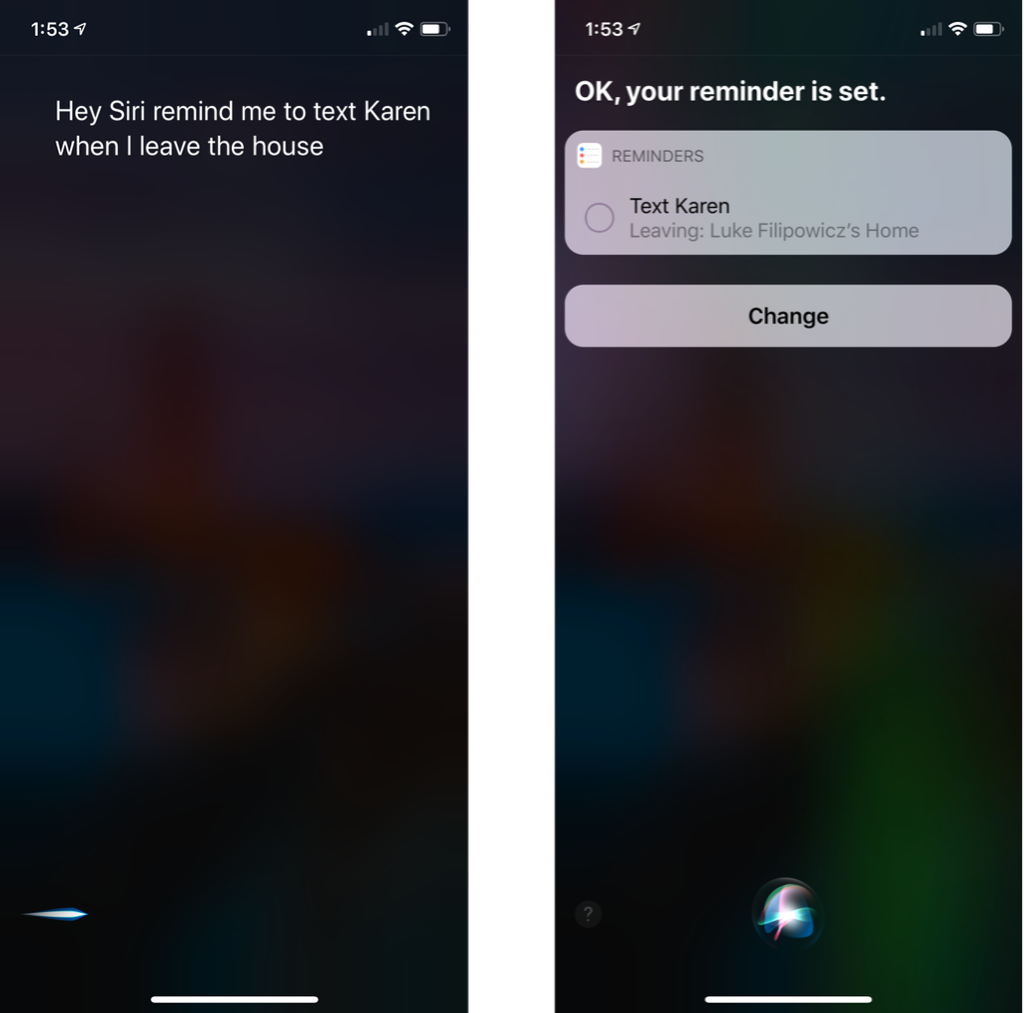The dual-image screenshot displays two side-by-side representations of a smartphone screen, specifically capturing a Siri interaction. Both screenshots show identical timestamps at 1:53, and feature various standard indicators in the status bar such as signal strength (displayed at one bar), full Wi-Fi signal, and a battery level at three-quarters full.

On the left screenshot, a user's Siri command is visible, saying, "Hey Siri, remind me to text Karen when I leave the house." The right screenshot illustrates Siri's response: "OK, your reminder is set."

Below the Siri responses on both screenshots is a light gray rectangle featuring a list of highlighted reminders. The list includes a reminder with a checkable box beside it, stating "Text Karen," followed by a specification, "Leaving: Luke P-O-W-I-C-Z’s Home." A "Change" button is also visible within this area. The reminders' list includes small, colorful bullet points in blue, red, and another color, adding visual organization to the tasks.